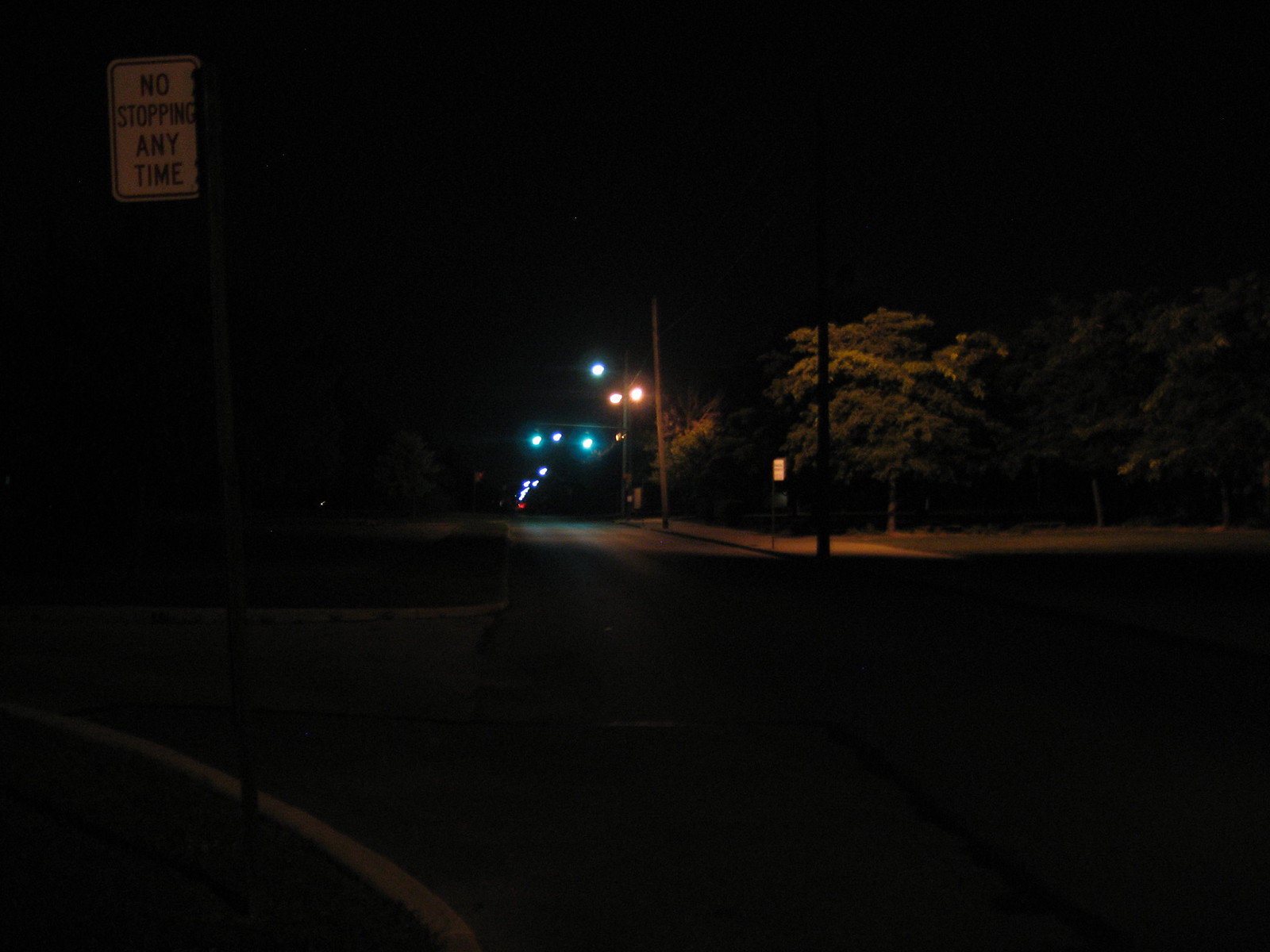This is a detailed color photograph taken at night, capturing a dark city street scene. The majority of the image is shrouded in darkness, with the foreground almost entirely black and barely visible. In the top left-hand corner, a dimly lit street sign reads "No Stopping Any Time," with black letters on a white background. The street extends into the background, where a variety of street lights create a poignant urban atmosphere. Two of these lights shine green, two emit an orange glow, and the rest radiate white. In the far distance, a red light - possibly a traffic signal or brake lights from a distant vehicle - is visible as a tiny dot. 

On the right side of the photo, near the foreground, stands a pole, behind which some partially lit green trees can be seen. The street itself lacks any visible line markings, suggesting it might be a two-lane road. A sidewalk follows along the right side, further dividing the street from the tree area. Above the street, you might catch a few stars in the night sky, adding a subtle celestial touch to the urban night scene. There are no cars on the road, emphasizing the serene and almost deserted feel of the night.